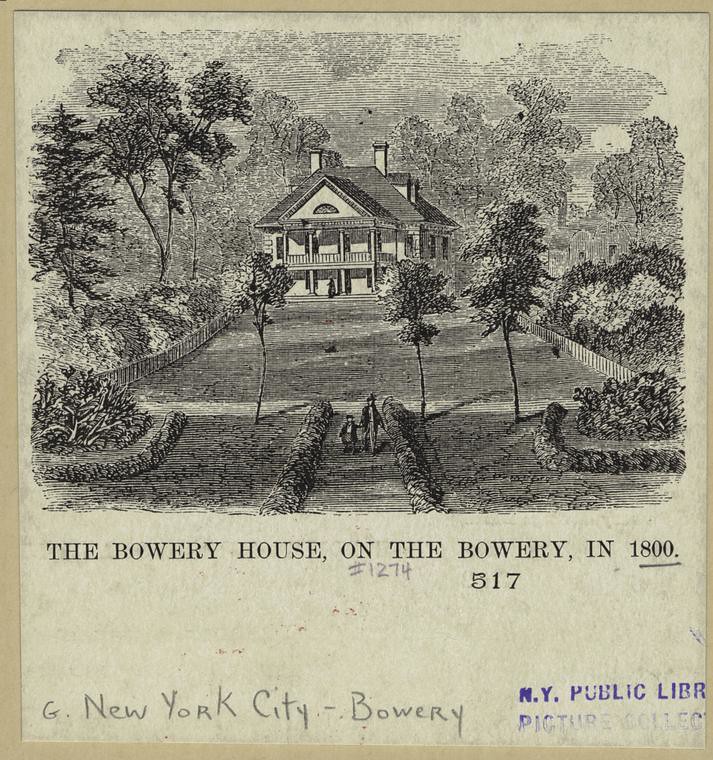This is a black-and-white photograph of "The Bowery House on the Bowery in 1800," from the New York City Public Library Picture Collection. The detailed image reveals a large, two-story house with an old-fashioned, plantation-like design, surrounded by bushes and trees. The photograph, which appears to be in an art print format, is bordered by a tan frame that complements its vintage aesthetic. In the bottom left corner, it is marked "New York City Bowery." Subtle hues of tan, off-white, black, gray, and a touch of bluish-purple add depth to the historical ambiance. Upon close examination, small figures of people can be seen at the lower part of the picture, adding a sense of scale and life to the serene setting, completed with an overall style that suggests its archival origin from the public library.